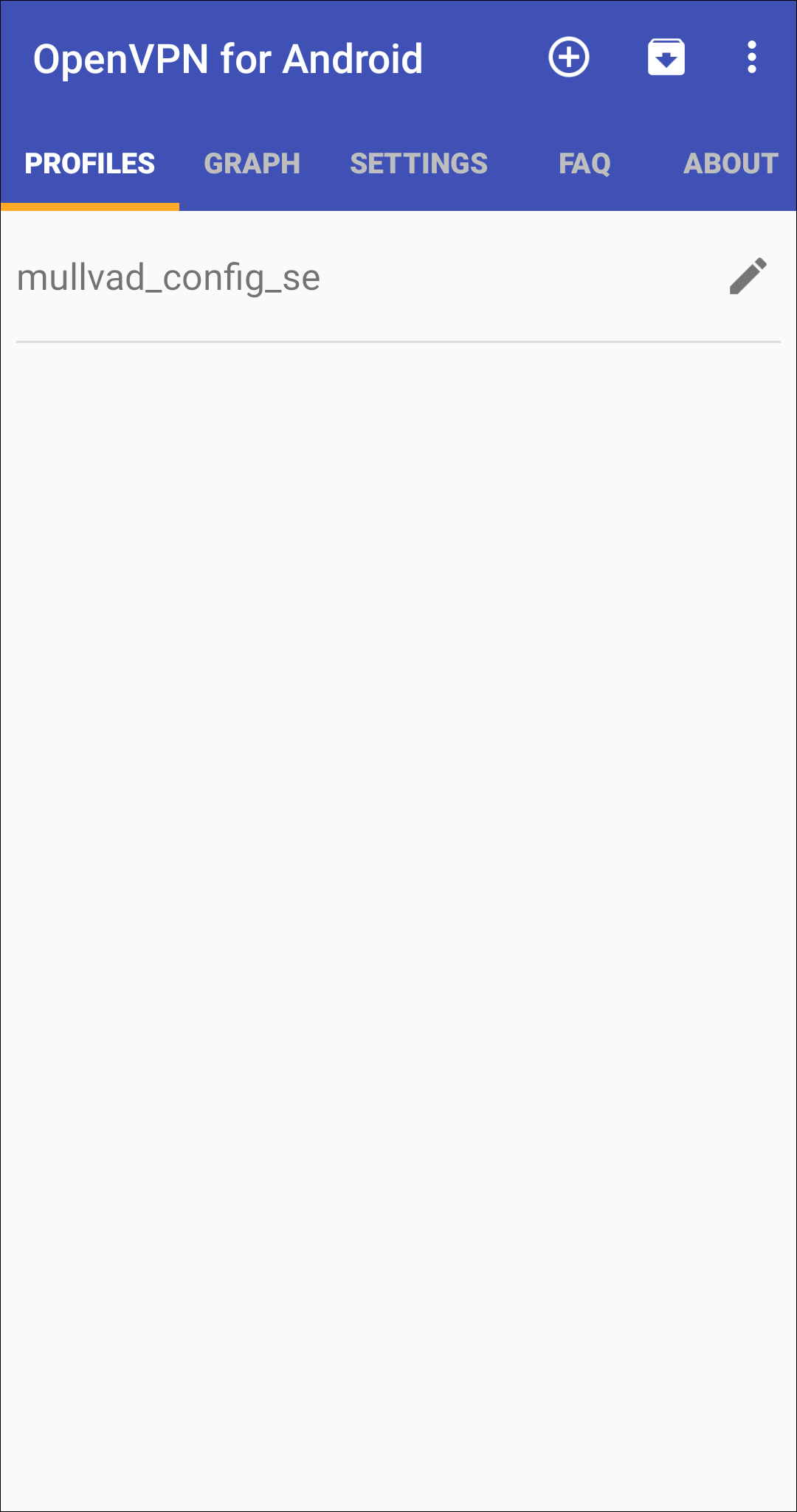This image showcases the OpenVPN for Android interface. The screen is predominantly white with accents of blue and gray. In the upper section, tabs labeled "Profiles," "Graph," "Settings," "Frequently Asked Questions," and "About" are visible. Below the tabs, a profile named "malvard_config_se" is listed. To the right of this profile, there is an edit button indicated by a small icon. Additionally, the interface includes various action buttons: an add or plus icon for creating new profiles, a download button, and a menu button for accessing more options. The overall layout is clean and user-friendly, adhering to the app's standard color scheme of blue, gray, and white.